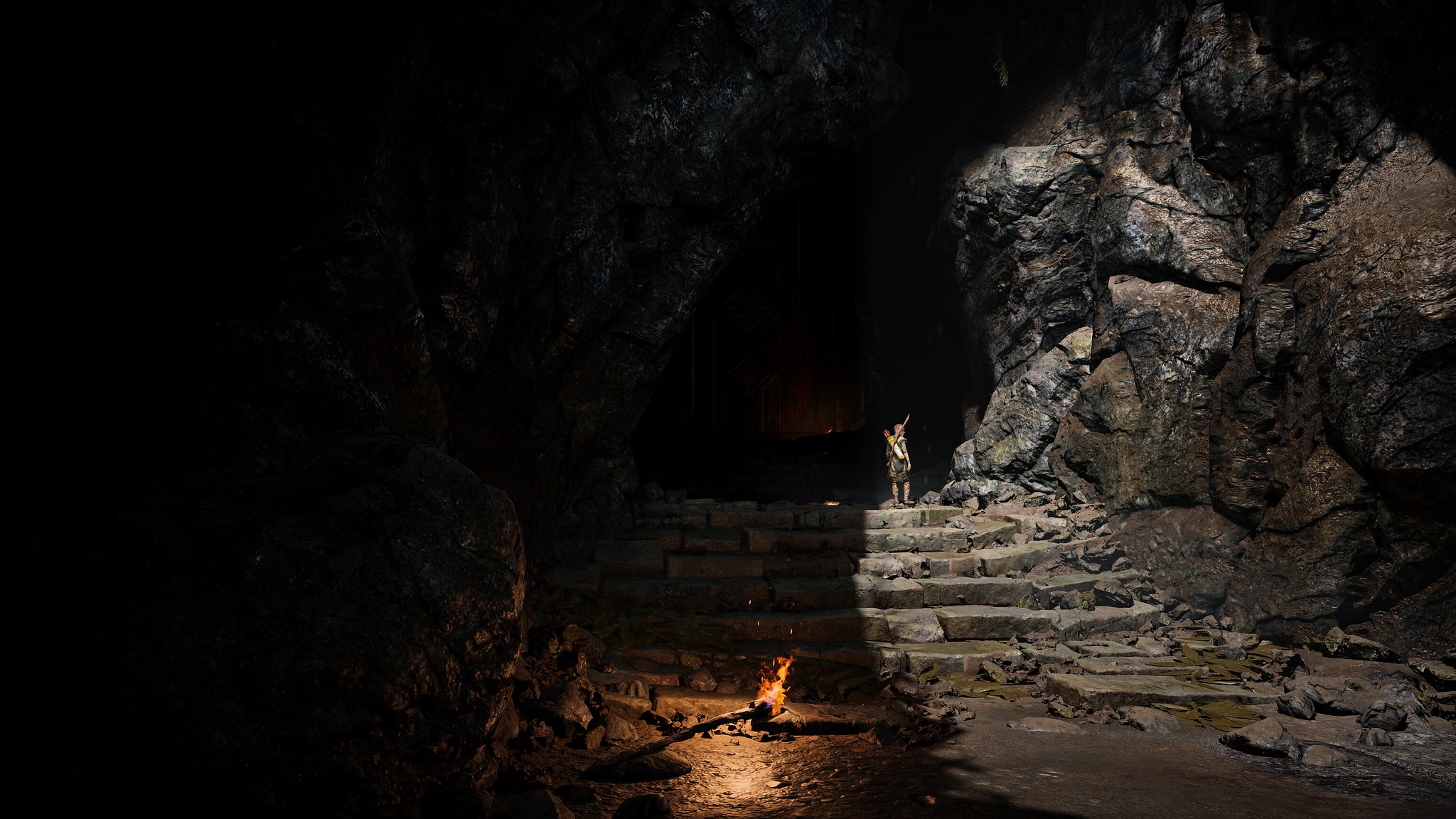The image depicts a highly detailed scene that appears to be from a modern video game, set within the dark, shadowy interior of a vast cave or canyon. The left side of the image is engulfed in darkness, while the right side is partially illuminated by sunlight peeking in from the top right corner, casting light on the rugged, gray rock formations. In the middle of the scene, at the base of a primitive-looking stone staircase, sits a small fire with orange and red flames, possibly from a dropped torch or small campfire, shedding limited light on its surroundings. Ascending the stone steps is a solitary figure, likely the game's playable character, with their back turned to the camera. This character appears to be a young person, clad in green clothing and a dress-like garment, carrying a bow and arrow along with a quiver strapped to their back. The overall ambiance of the image is dark and mysterious, with intricately textured stone walls and a sense of adventure and exploration.